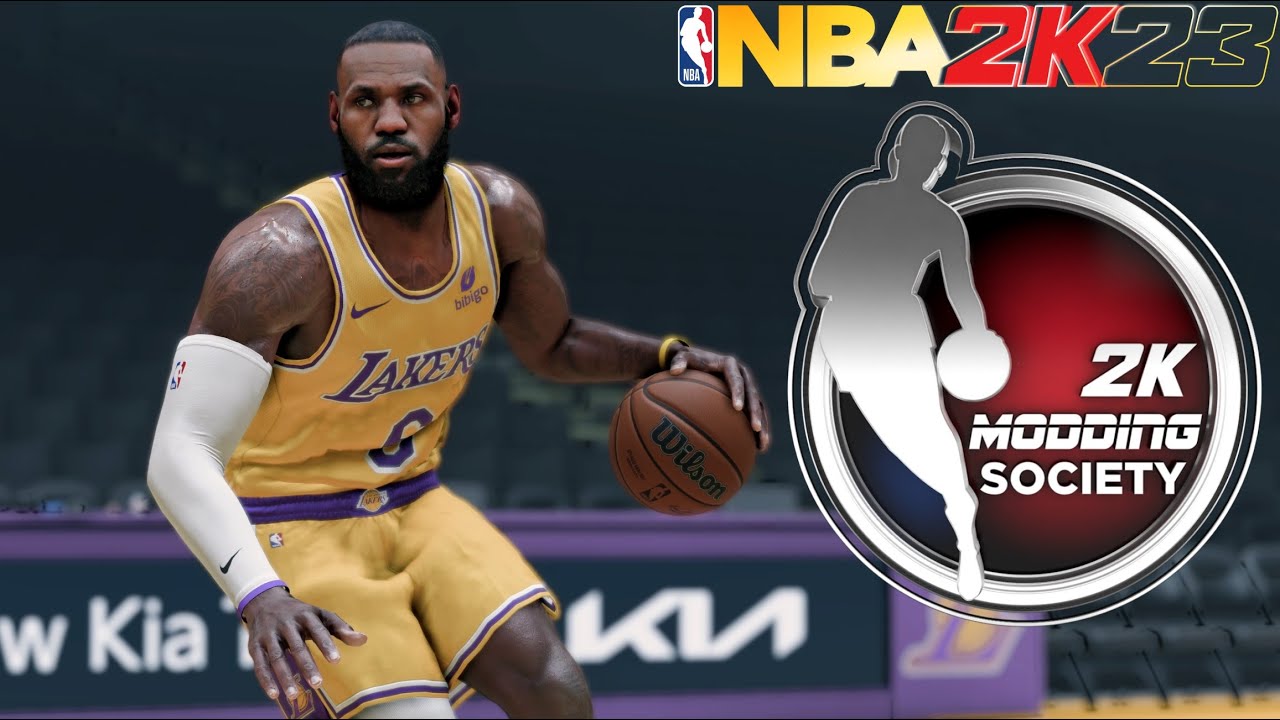In this image, LeBron James is captured in mid-action, poised to dribble the basketball. He dons his iconic Los Angeles Lakers uniform, a vibrant yellow ensemble with "Lakers" emblazoned in purple across the chest. Although the uniform number is obscured, the setting is unquestionably immersive, placing James on a basketball court towards the left center of the frame.

To the right in the upper portion of the image, branding elements of the basketball video game series 'NBA 2K' are prominently displayed. The text reads "NBA" in yellow, "2K" in red, and "23" in black; all positioned next to the classic NBA logo which features red, white, and blue colors.

Below these elements lies another graphic, showcasing the "2K Modding Society" emblem. This insignia is a silver circle with the text "2K Modding Society" written in white around its inner edge. The circle's interior background is a reddish-maroon hue, and on its left is an adjacent, somewhat interrupted image of a figure holding a basketball, seamlessly integrating into the badge's design.